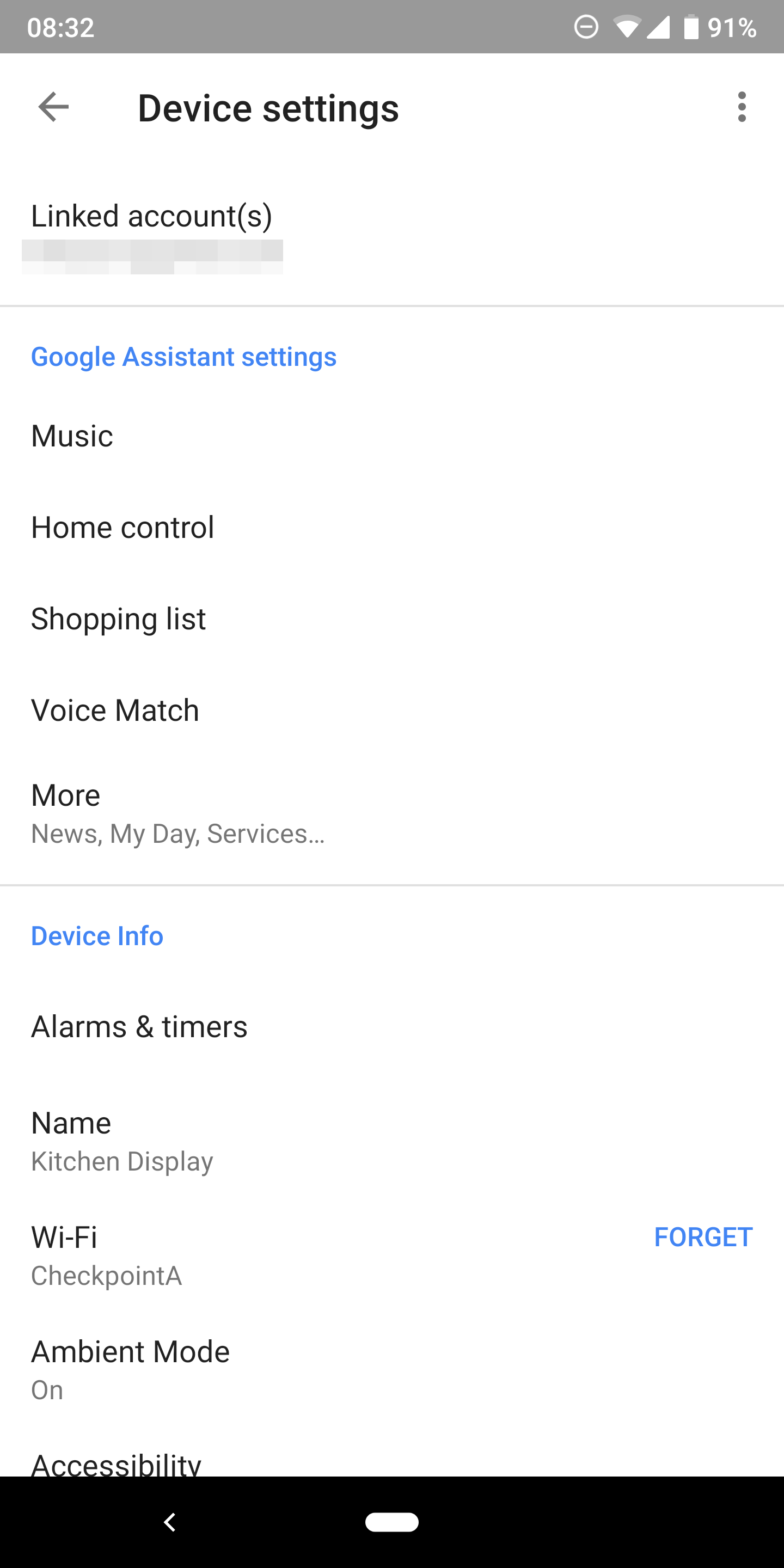The image appears to be a screenshot from a mobile device, specifically displaying a settings menu for Google Assistant. At the very top, there is a slim grey bar where the left corner shows the time as 8:32. To the right of the time, there are icons indicating the Wi-Fi signal strength, battery status, and battery percentage at 91%.

Below this bar, the screen transitions to a white background where the first heading, “Device Settings,” is prominently displayed. Under this heading, the option "Linked Accounts" is present but grayed out, indicating it may not be accessible at this time. 

Further down, another heading in blue reads, "Google Assistant Settings." This section includes several options: "Music," "Home Control," "Shopping List," "Voice Match," and an option labeled "More." Under the "More" section, additional items listed are "News," "My Day," and "Services."

A grey line divides this section from the next, where the heading "Device Information" appears in blue. This part of the screen contains options for "Alarms and Timers," and "Name," which appears as "Kitchen Display." The Wi-Fi settings indicate the current network as "Checkpoint A," with an option to the right labeled "Forget" in blue. The section also mentions "Ambient Mode On" and "Accessibility."

At the very bottom of the screen, a black band is visible with a small triangle pointing left, and a white rectangle positioned centrally, likely representing the home and navigation controls of the device.